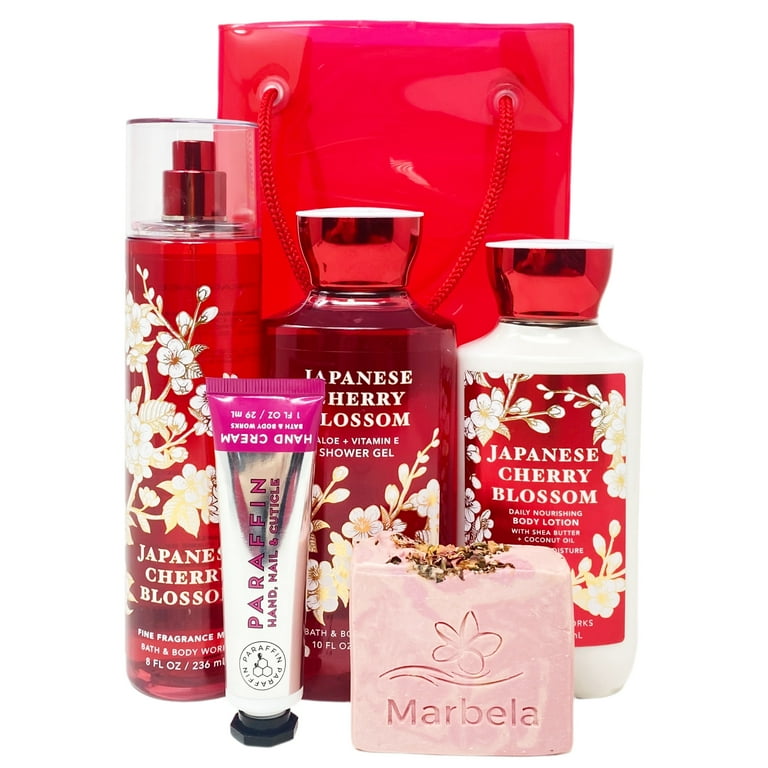This detailed and cohesive caption for the image incorporates elements from each initial description, focusing on shared and repeated details:

---

The image showcases an elegant gift set designed for bathing and hygiene, prominently featuring a red and white color scheme. Anchoring the display in the background is a shiny red gift bag with a red rope handle. There are three vertical containers labeled "Japanese Cherry Blossom" that exude a coordinated aesthetic. On the left, a circular spray container with a transparent cover reveals a red liquid. Centered in front is a sleek tube of hand cream, also labeled "paraffin, hand, nail, and cuticle," balanced on its black cap. Nestled beside it is a sophisticated bar of soap, pinkish-white in tone, engraved with "Marabella" and adorned with delicately carved curvy lines and flower petals. Two oval-shaped bottles flank the soap: one containing a red liquid shower gel and the other, a body lotion, also adorned with white flowers and labeled "Japanese Cherry Blossom." Together, these items compose a luxurious set perfect for gifting.